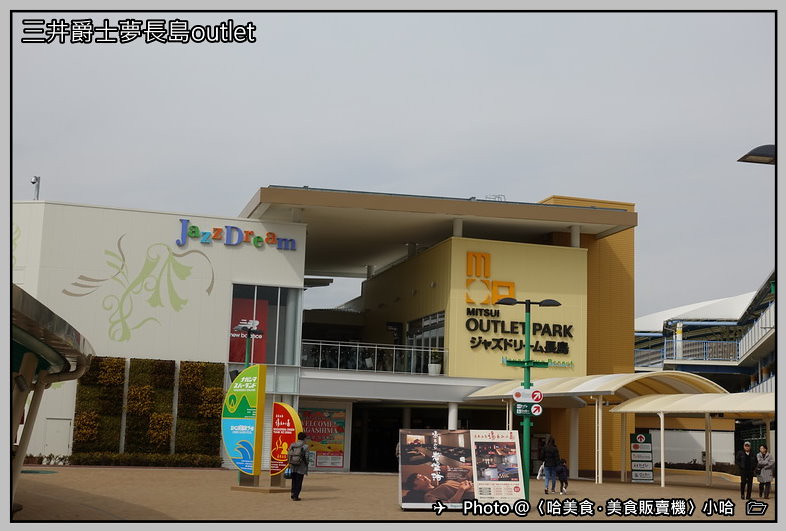The image depicts the bustling exterior of Mitsui Outlet Park, a modern shopping mall with a vibrant facade primarily painted in yellow and white. Prominently featured is the text "Jazz Dream" in colorful blue, green, and red letters on the left side of the building, accompanied by a floral decoration on a white background. Below the main signage, foreign characters likely translating "Mitsui Outlet Park" are visible. The architecture showcases modern design elements, including a two-storey structure with an awning-covered walkway leading to the mall's interior, designed to protect visitors from the rain. Various billboard advertisements in vibrant red, yellow, green, and blue are strategically placed on the front and windows of the mall, promoting different stores within. In the foreground, a well-dressed couple in suits and coats is seen exiting from the right side, while a woman with a child and a man carrying a backpack are heading towards the entrance, highlighting the mall's active and inviting atmosphere.